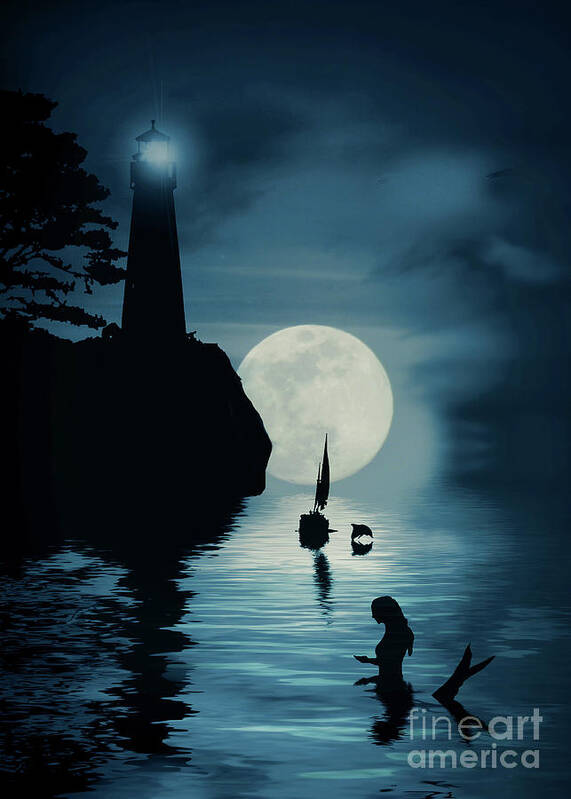In this detailed computer-generated artwork set during a dark, oceanic night, the focal points include a dark blue ocean with lighter blue gradients closer to the center, and a full moon illuminating the scene. On the left, a lighthouse stands on a cliff with its beams cutting through the night, and adjacent to it, a tree with visible leaves. In the ocean's foreground on the right, a mermaid is partially emerged from the water, revealing her human-like torso and fish-like tail. Behind her, a small boat recedes into the distance with a dolphin leaping nearby. The bottom right corner bears the text "Fine Art America."